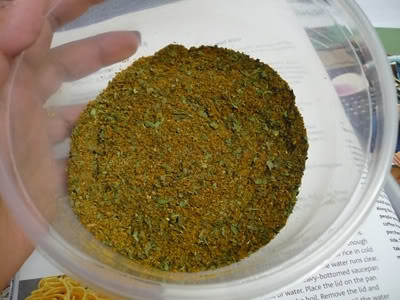A photograph showcases a hand, likely female, holding a clear bowl filled with a mixture of dry spices. The mixture, primarily orange and brown in hue, includes visible green herb leaves, perhaps oregano or basil, along with faint specks of yellow spice, resembling breadcrumbs or dried parsley. The translucent bowl reveals the holder's hand and is positioned over an open book, likely a cookbook. The book's white pages with black text are visible, and in the bottom left corner of the book, there's an image of spaghetti, reinforcing the culinary context. In the background, a green object and a calculator can also be seen.